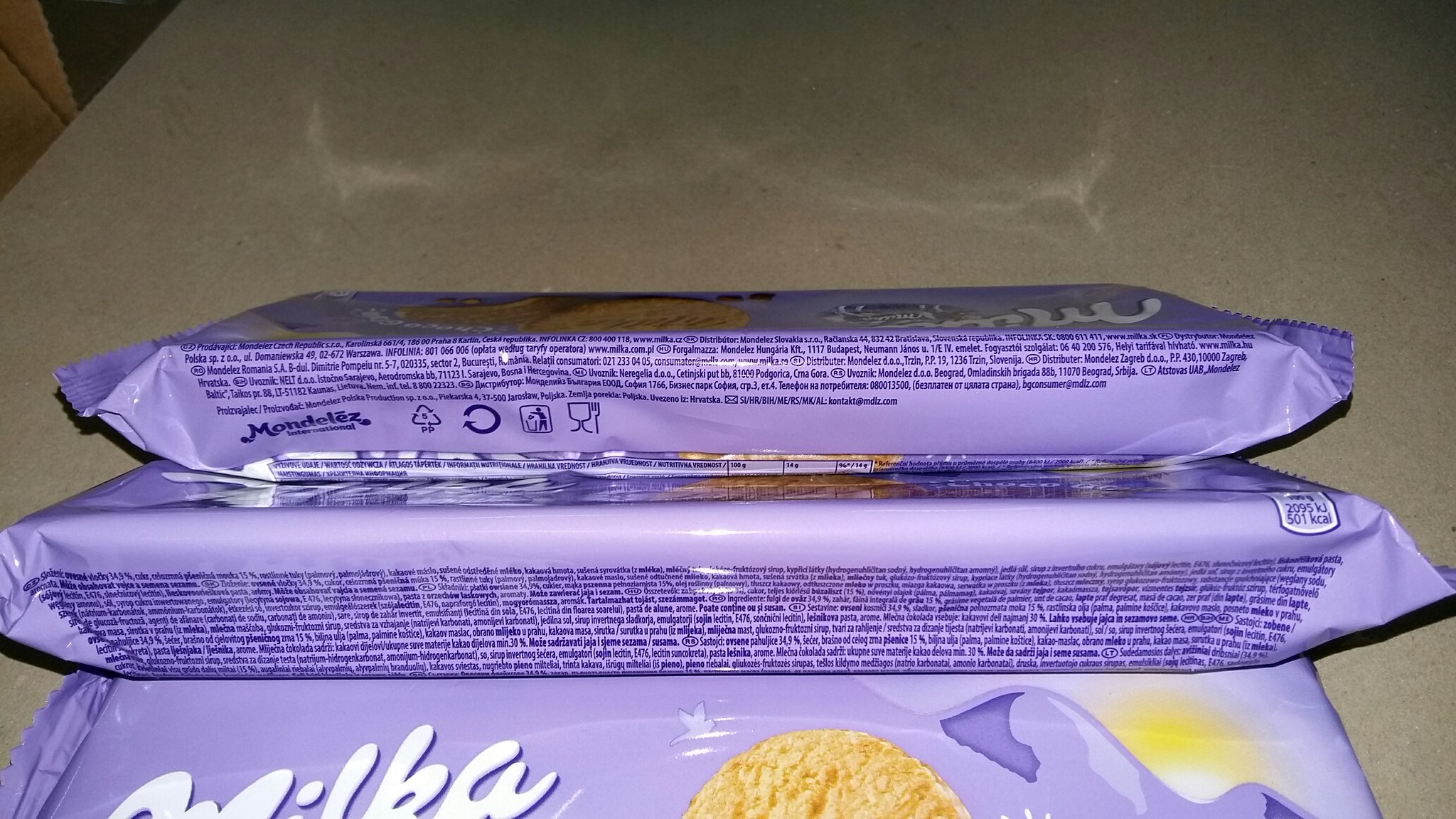This photograph, slightly dark with moody lighting, showcases three snack packages, likely cookies, on a gray countertop that features some white, cloudy areas. The image spans about one and a half times wider than it is tall, with the snacks positioned predominantly in the lower two-thirds to three-quarters of the frame. The packages themselves are light purple, bearing the brand name "MILKA" in white letters, partially obscured but visible on the package lying flat.

This package, which lies with its greater area facing up, shows part of a cookie image to the right, alongside what appears to be a small sun and mountain motif. Flanking this flat package, the other two are propped diagonally against it, exposing their shorter sides. These sides are densely printed with lines of text listing ingredients, with one bearing extra branding details, including the name "Mondelez" in the lower right corner. The composition of the packages, their pastel color, and the intricate text detail focus bring a structured yet casual presentation of everyday snack items to life.